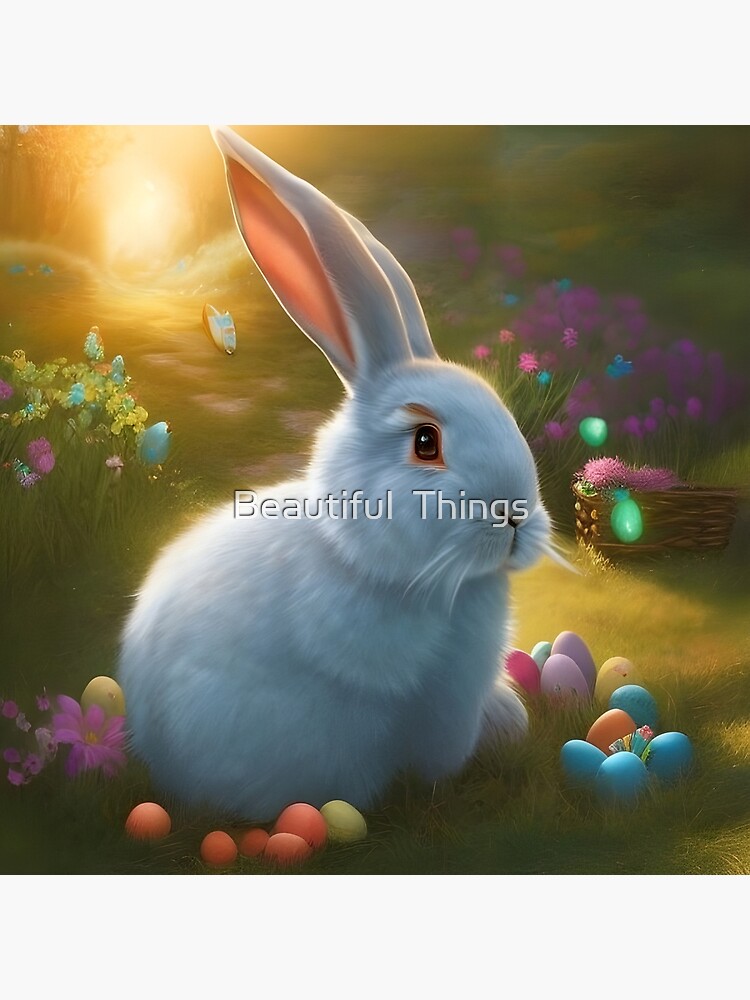This digital artwork, potentially AI-generated, depicts an Easter-themed scene centered around a fluffy white rabbit with long ears that have pink or red centers. The rabbit, sitting upright with its legs tucked in, appears almost ball-like and is positioned in the middle of the image. It has a single black eye accented with red and brown hues, white whiskers, and large dark brown eyes. Surrounding the rabbit are an array of colorful Easter eggs—red, yellow, blue, purple, pink, and green—distributed on the ground and even floating above a wicker basket to the rabbit's right. Numerous flowers in pink, purple, blue, and yellow adorn the scene, particularly on the left side and along a trail in the background. A bright, glowing light, presumably the sun, illuminates the horizon atop a distant hill on the left, casting an overall warm and festive ambiance. The artist's name, spelled A-N-Y-T-K-A, is prominently displayed over the rabbit, adding an additional layer of intrigue to this enchanting Easter depiction.